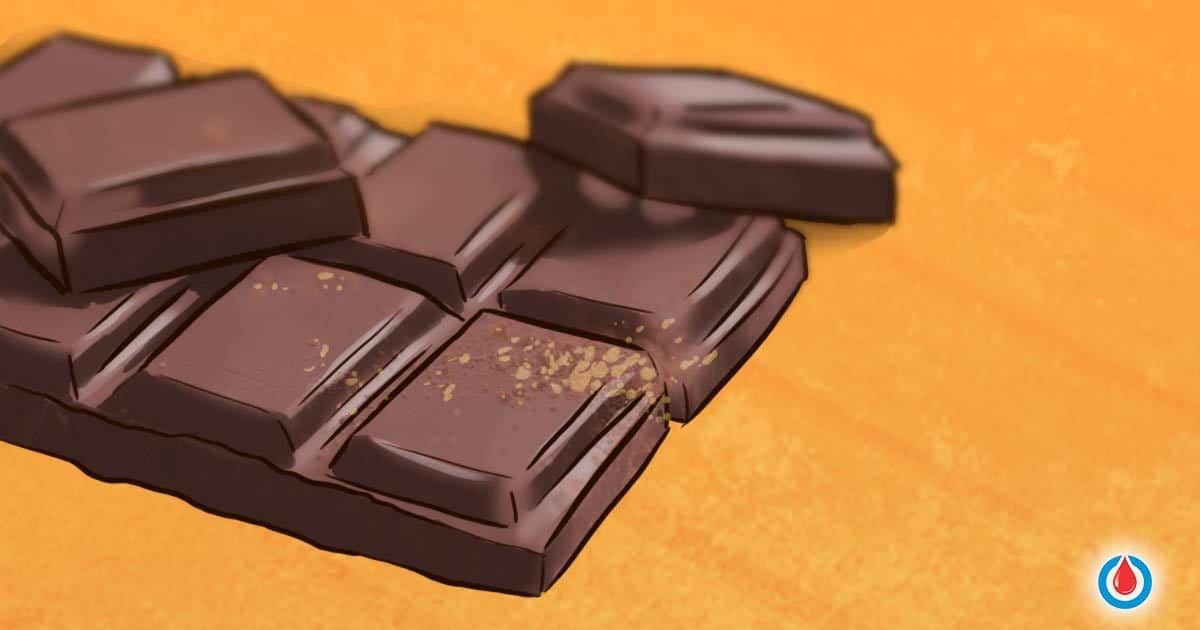A highly realistic sketched chocolate bar takes center stage in this detailed graphic illustration. The bar, depicted in rich brown hues, is positioned against a rustic, jewel-toned orange background that evokes the warmth of an autumnal pumpkin. This inviting backdrop, devoid of distractions on the right-hand side, draws the viewer's focus to the chocolate bar, which extends from the left into the center of the image. 

The chocolate bar features seven visible squares in a two-by-four formation, with additional squares broken off. One broken piece rests on top of the bar towards the left, while another leans off the edge towards the right, creating a dynamic and natural arrangement. A subtle dusting of cocoa powder enhances the bar's texture, adding to its visual allure. The artist's skillful rendering leaves ambiguity as to whether the piece is hand-drawn or digital art but is undeniably detailed and realistic.

Additionally, in the lower right-hand corner, there is a logo featuring a distinctive red raindrop encased in a blue circle, adding a unique element to the composition.